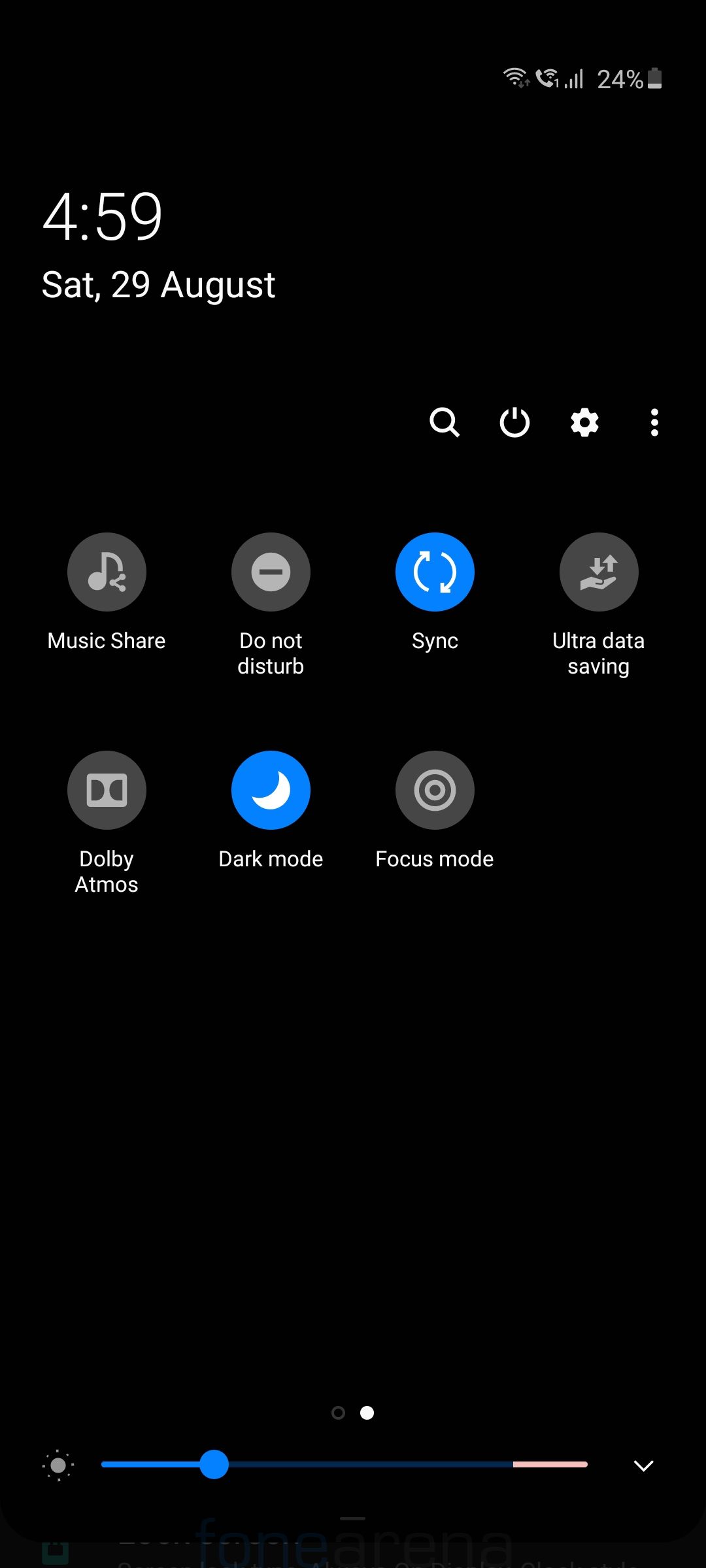The screenshot of the mobile device captures a detailed view of the status bar at the top of the screen. In the top right corner, a fully illuminated Wi-Fi signal icon indicates a strong connection, displaying all 4 out of 4 bars. Adjacent to the Wi-Fi signal, a voice-over Wi-Fi icon confirms the device's capability for internet-based calls. Next, the network signal strength is also at its peak, with all 4 bars filled. Moving further right, the battery percentage is critically low at just 4%, marked by a noticeable red color.

Additionally, the status bar is populated with several icons representing active features and modes. The Do Not Disturb icon implies notifications and alerts are silenced. The Sync symbol indicates that data synchronization is currently engaged. Ultra Data Saving mode is active, suggesting measures are being taken to conserve mobile data. Even the Dolby Atmos icon is present, hinting that enhanced sound settings are enabled. The Dark Mode icon confirms that the device is set to a dark theme, likely to reduce eye strain and save battery life. Focus Mode is turned on, aiding in minimizing distractions. Lastly, the Music Share icon shows that the device is set to share audio with other Bluetooth devices.

This meticulous snapshot conveys comprehensive information about the device’s current status and active settings, all in one glance.